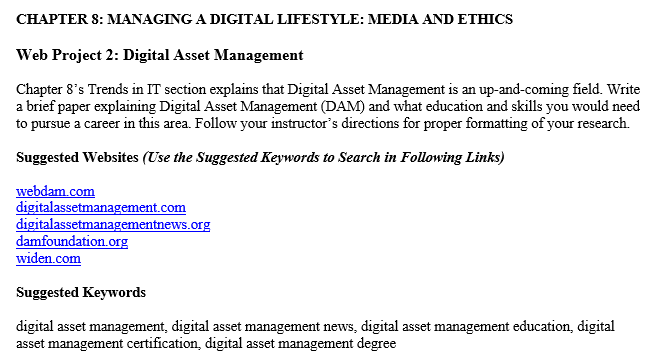The image appears to be an instructional section from an educational resource, possibly a textbook or an online course module. It features Chapter 8 titled "Managing a Digital Lifestyle: Media and Ethics," with the title prominently displayed in bold, all-uppercase black text.

Below the chapter title, there is a heading for "Web Project 2: Digital Asset Management," where "Web Project 2" and "Digital Asset Management" are capitalized, emphasizing the importance of the assignment.

The content under Chapter 8 details trends in Information Technology (IT) with a specific focus on the emerging field of Digital Asset Management (DAM). The text prompts the reader to write a brief paper explaining what Digital Asset Management entails and outlines the educational background and skills necessary to pursue a career in this domain. The acronym "DAM" is highlighted, with each letter capitalized to distinguish its importance.

Students are instructed to follow their instructor's guidelines for formatting their research paper properly. Suggested websites for further research are listed, including:
- webdam.com
- digitalassetmanagement.com
- digitalassetmanagement.org
- damfoundation.org
- widen.com

Additionally, suggested keywords to use in searches are: "digital asset management," "digital asset management news," "digital asset management education," "digital asset management certification," and "digital asset management degree." These keywords are intended to help students find relevant information and resources.

The image is likely an assignment page, providing detailed instructions for a web project focused on Digital Asset Management within the context of managing a digital lifestyle and understanding media ethics.